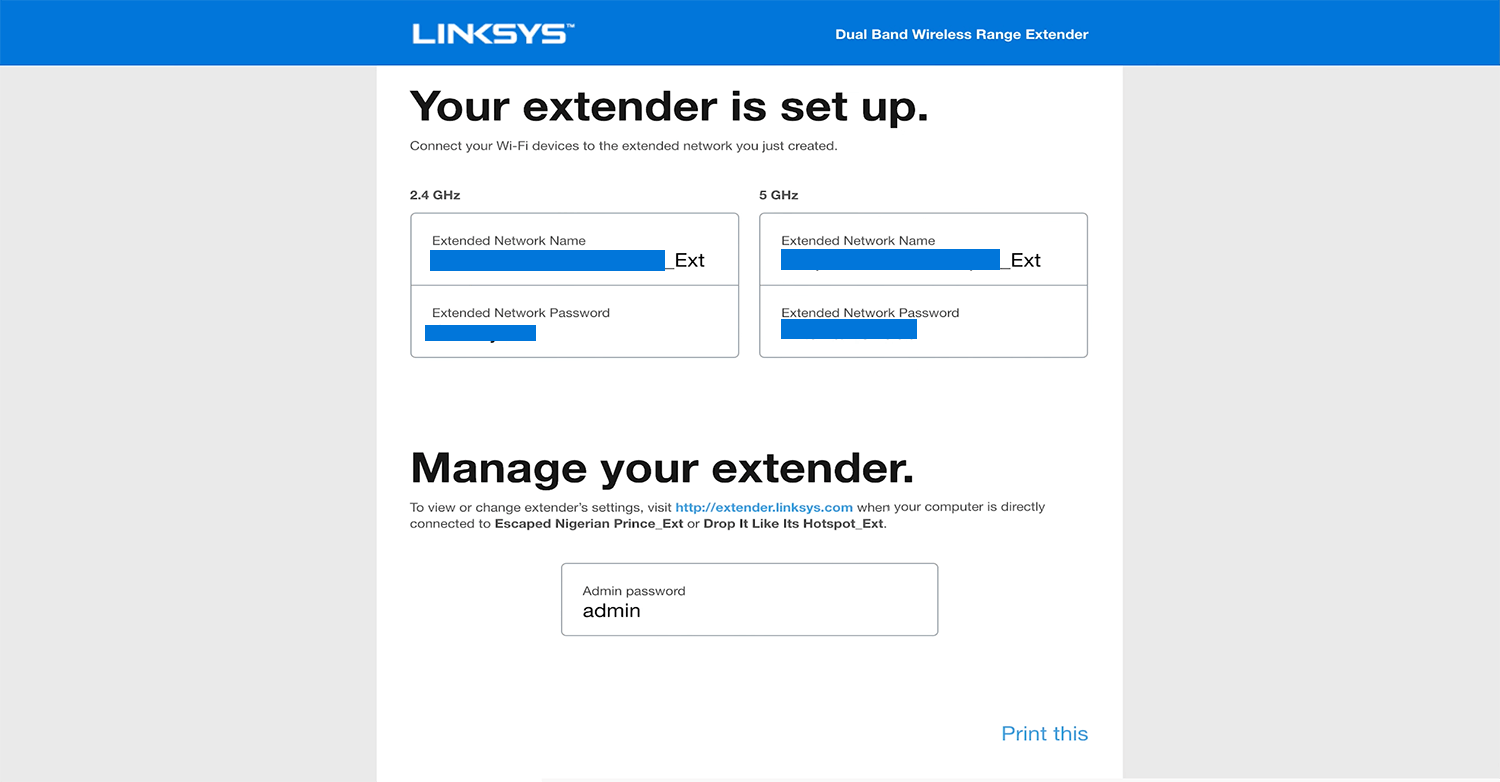This screenshot captures the configuration page of a Linksys Dual-Band Wireless Range Extender on their official website. The header features a distinct blue bar with the "LINKSYS" logo prominently displayed in all capital white letters. To the right of the logo, it specifies the product as a "Dual Band Wireless Range Extender."

Below the header, the page indicates that "Your extender is set up." It prompts the user to connect their Wi-Fi devices to the newly created extended network. The page provides two options for network settings:

1. **2.4 GHz Extended Network:**
   - **Extended Network Name:** Displayed with a blue rectangular box obscuring the actual network name.
   - **Extended Network Password:** Also hidden under a blue rectangular box.

2. **5 GHz Extended Network:**
   - **Extended Network Name:** Similarly, this is concealed by a blue rectangular box.
   - **Extended Network Password:** Again, hidden under a blue rectangular box.

Additionally, the page offers instructions to manage the extender: "To view or change extender settings, visit extender.linksys.com when your computer is directly connected to ESCAPE_NIGERIAN_PRINTS_extension or drop_it_like_its_hot_extension. The admin password is 'admin'."

In the bottom right-hand corner of the page, there is a link labeled "Print this" in blue lettering.